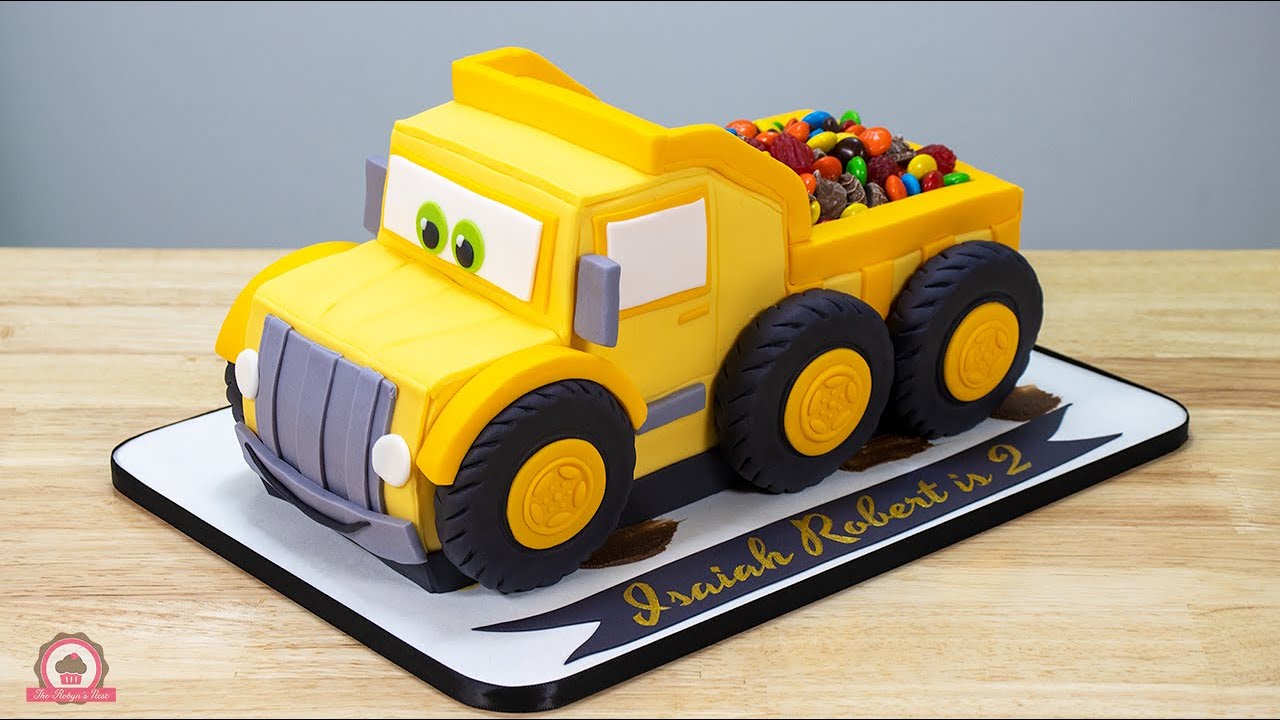This image showcases a meticulously crafted birthday cake designed to resemble a toy dump truck, likely made for a boy's second birthday celebration. The bright yellow truck cake is enhanced with cartoon-like features, including a gray grille, two green eyes on the front windshield, and white windows. The truck is set on a white serving tray with black trim, which rests on a light brown wooden table against a gray wall backdrop. Notably, the serving tray bears the cursive inscription "Isaiah Robert is two." The truck's rear bed is filled with colorful candy pieces such as M&Ms or Skittles. The truck has three black tires with yellow rims visible on one side, adding to its playful and charming appearance. In the bottom left corner of the image, a small logo resembling a cupcake with a pink wrapper and brown icing adds a distinctive bakery touch.